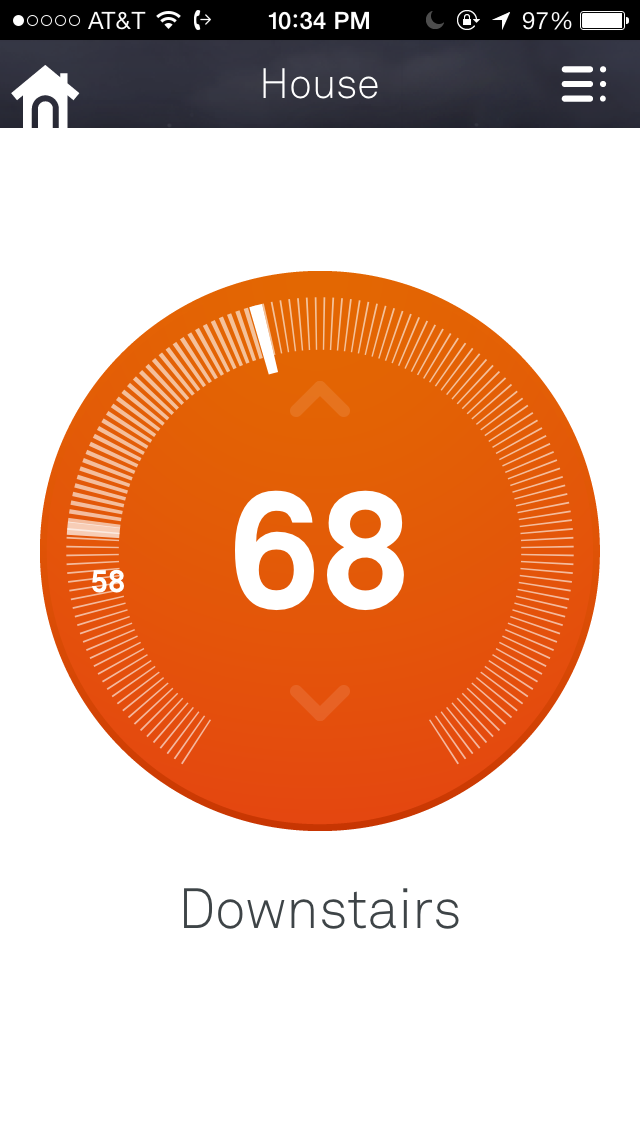The image depicts a Nest thermostat interface as it appears on a smartphone screen. The main focus is an orange circular dial prominently displaying the temperature set at 68°F in large white numbers at its center. Surrounding the dial are numerous small white tick marks, with a darker tick indicating the current temperature setting. Below the number 68 is a faint, upside-down chevron pointing downward, while a similar chevron is located above the number, likely functioning as touch controls to adjust the temperature.

To the right of the orange dial, a smaller number 58 is visible, though its significance remains unclear. At the top  of the interface, there is a black stripe displaying various status icons and information. This includes the label "AT&T," a strong Wi-Fi signal indicator, and a telephone icon with an arrow pointing right. The current time is shown as 10:34 PM, accompanied by a small moon icon indicating nighttime. Additional elements on this stripe include a circular icon with a closed padlock, a small upward-pointing arrow, a battery icon indicating a 97% charge level, and a house icon on the left. In the middle is the word "House," and towards the right is a hamburger menu with three lines, followed by three dots.

The combination of these details indicates that the screen is likely part of a smartphone app used to control and monitor the Nest thermostat remotely, managing the home's heating and cooling system efficiently.